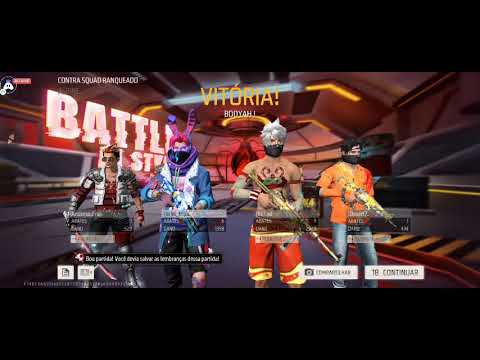The image is a pixelated, letterboxed screenshot from the video game Fortnite, featuring four characters standing side-by-side as if on a team selection screen. Each character is holding a weapon, with the first on the left wielding a katana sword. This character wears a silver vest over a red undershirt and has red hair and sunglasses. The second character sports a blue denim jacket, a purple scarf, pink bunny ears, a purple hood, and pink hair, holding a firearm—likely an assault rifle or shotgun. The third character, shirtless and covered in red tattoos, has white hair and a black face covering, and is equipped with a long golden and red gun. The final character on the far right is dressed in an orange shirt and blue jeans, with a black scarf covering the lower half of his face, holding a yellow assault rifle. They all stand in a red and brown hangar or tunnel background, with the word "battle" and the text "Vitoria!" visible in the scene.